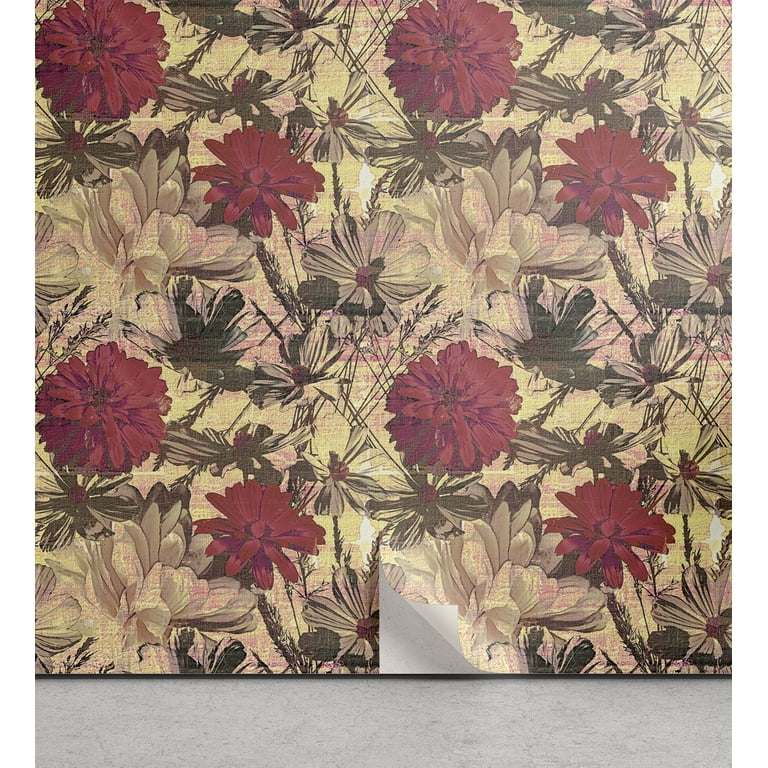The image depicts a floral wallpaper with a light yellow background adorned with a very busy and intricate pattern featuring multiple flowers. Dominating the design are large, dark red flowers resembling chrysanthemums that have many petals, and smaller flowers that vary in type, including white daisies with red centers and pale green and pink flowers. The wallpaper appears to be aged or damaged, as parts are peeling off, especially near the bottom where an entire corner is lifted, exposing the wall behind it. In this damaged area and also in spots further up, the wallpaper is either ripped or missing entirely. The floral imagery is complemented by green leaves interspersed among the flowers. The setting includes a floor that appears to be gray marble in front of the wallpaper.